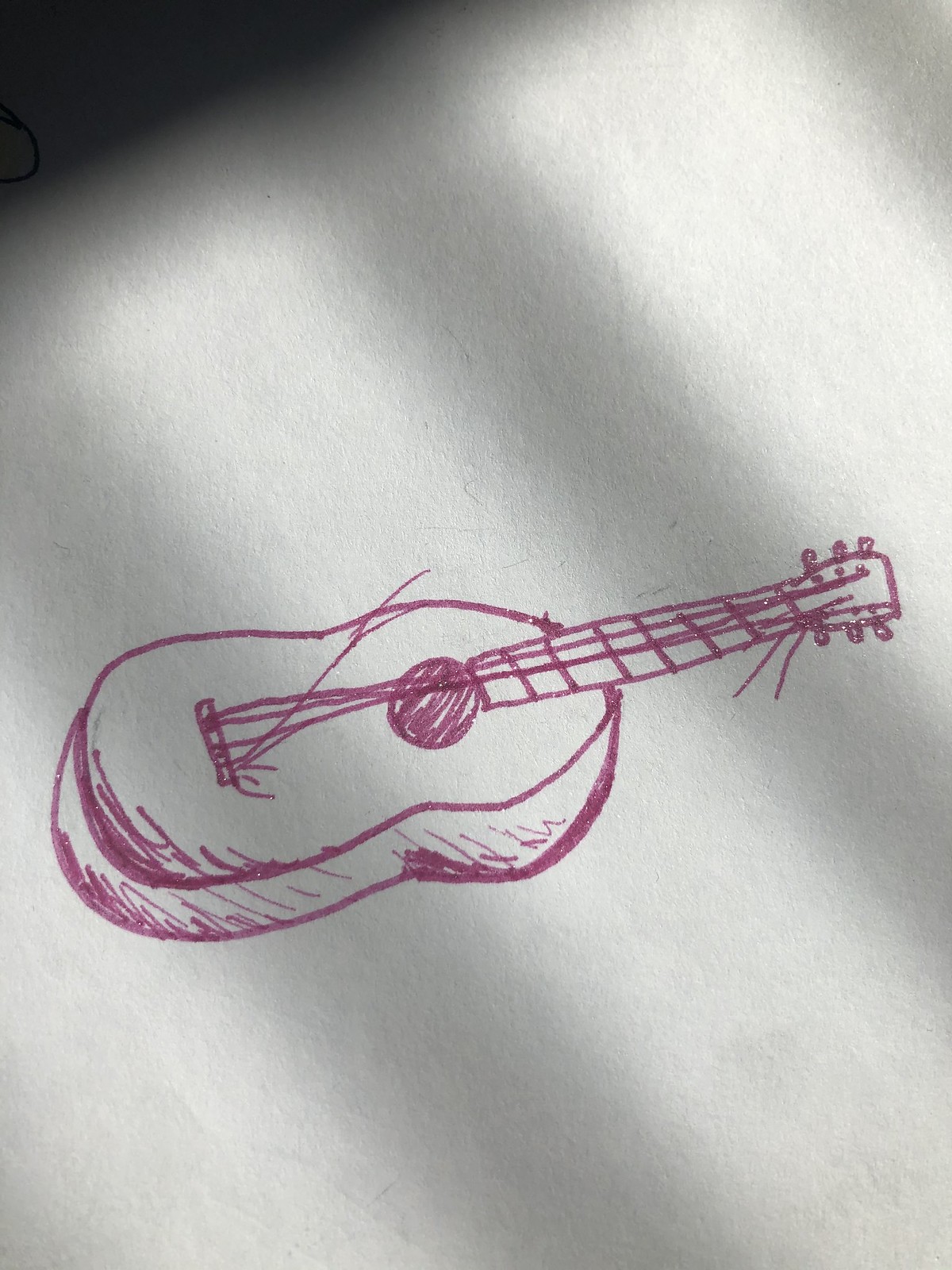The image is a detailed color sketch of an acoustic guitar, illustrated with a purplish-pink ink, possibly using a glittery gel pen. The guitar is drawn on a white surface, though the exact material (paper, stone, or wall) is not clearly identifiable. The sketch captures the traditional curvy shape of an acoustic guitar, complete with a central soundhole. Notably, several strings are depicted as snapped—some towards the bottom and some at the top of the neck—leaving only three strings intact, stretching from the bottom to the top. The guitar also features subtle shading on its left side, enhancing its dimensionality. There is a small shadowed area in the image's top left corner, possibly from the lighting, which suggests that the light source could be coming through window blinds. The overall perspective of the guitar's portrayal might appear slightly off, which adds a bit of a unique charm to the illustration.